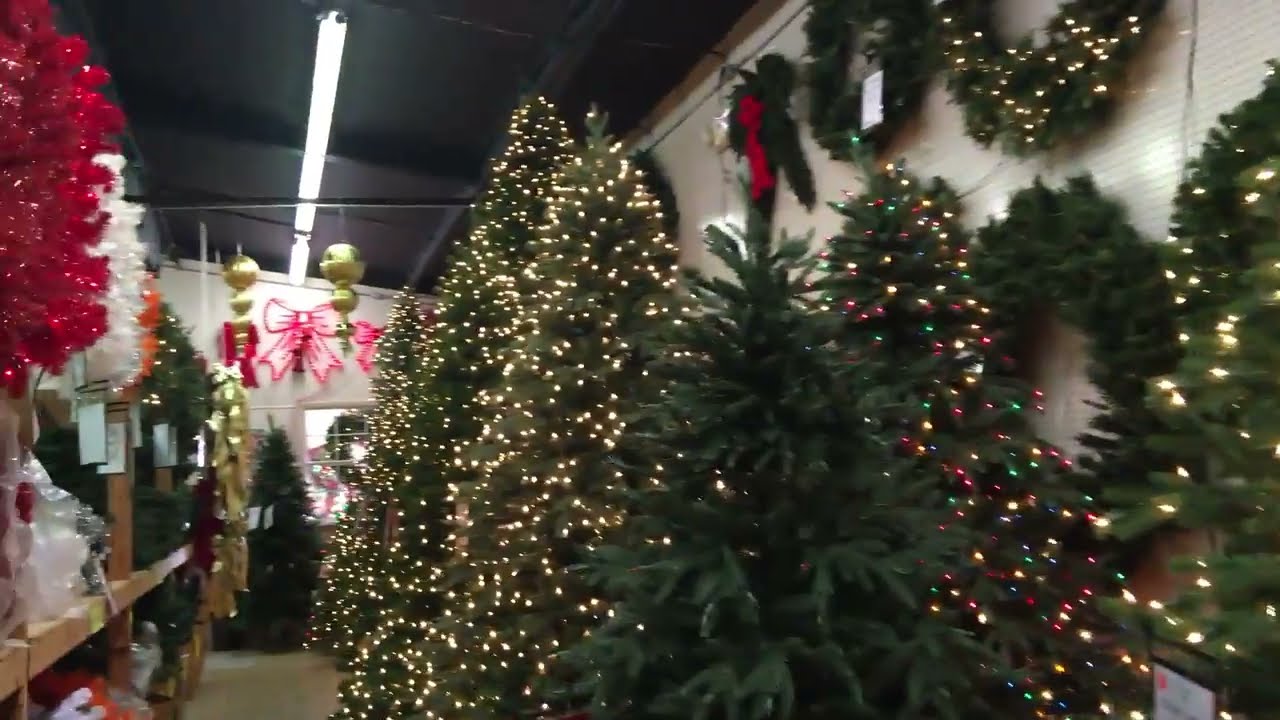This image captures the interior of a Christmas-themed shop adorned with numerous festive decorations. Dominating the scene are an array of artificial Christmas trees clustered in the middle and right side, some adorned with twinkling white lights and others festooned with colorful lights. The left side of the image features distinctly red and white trees. Surrounding these trees, the white walls host several wreaths; some are simple, while others are illuminated or embellished with red bows. Elevated on the left side is a wooden shelf displaying additional decorations, including tinsel and green foliage. The decorations extend to the high black ceiling, where bows and hanging ornaments add to the festive atmosphere. A prominent fluorescent light beams down, illuminating the white floor below. The background fades into more greenery, contributing to the dense, festive ambiance of the store.